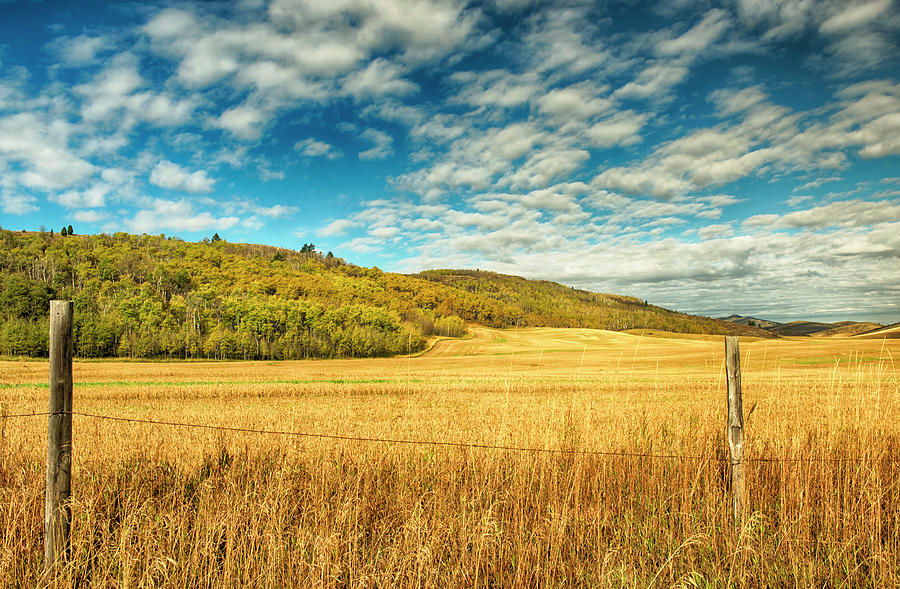This high-quality photo captures a serene, sunlit Midwest farmland scene. At the forefront, an old-fashioned wooden fence with barbed wire stretches between two wooden posts spaced approximately 10 to 12 feet apart. Beyond the fence lies a vast field of vibrant, golden-yellow wheat that appears almost luminous under the midday sun. The absence of shadows suggests the photo was taken around noon. In stark contrast to the dry, sun-bleached field, the background is filled with lush, green hills peppered with a mix of verdant and autumnal yellow trees, hinting at the fall season. Above, the sky is a stunning shade of blue, dotted with scattered, fluffy white clouds, adding to the peaceful ambiance of the scene. The vibrant colors of the landscape give it an almost amplified, lively appearance. No people or animals are present, highlighting the undisturbed beauty of nature.